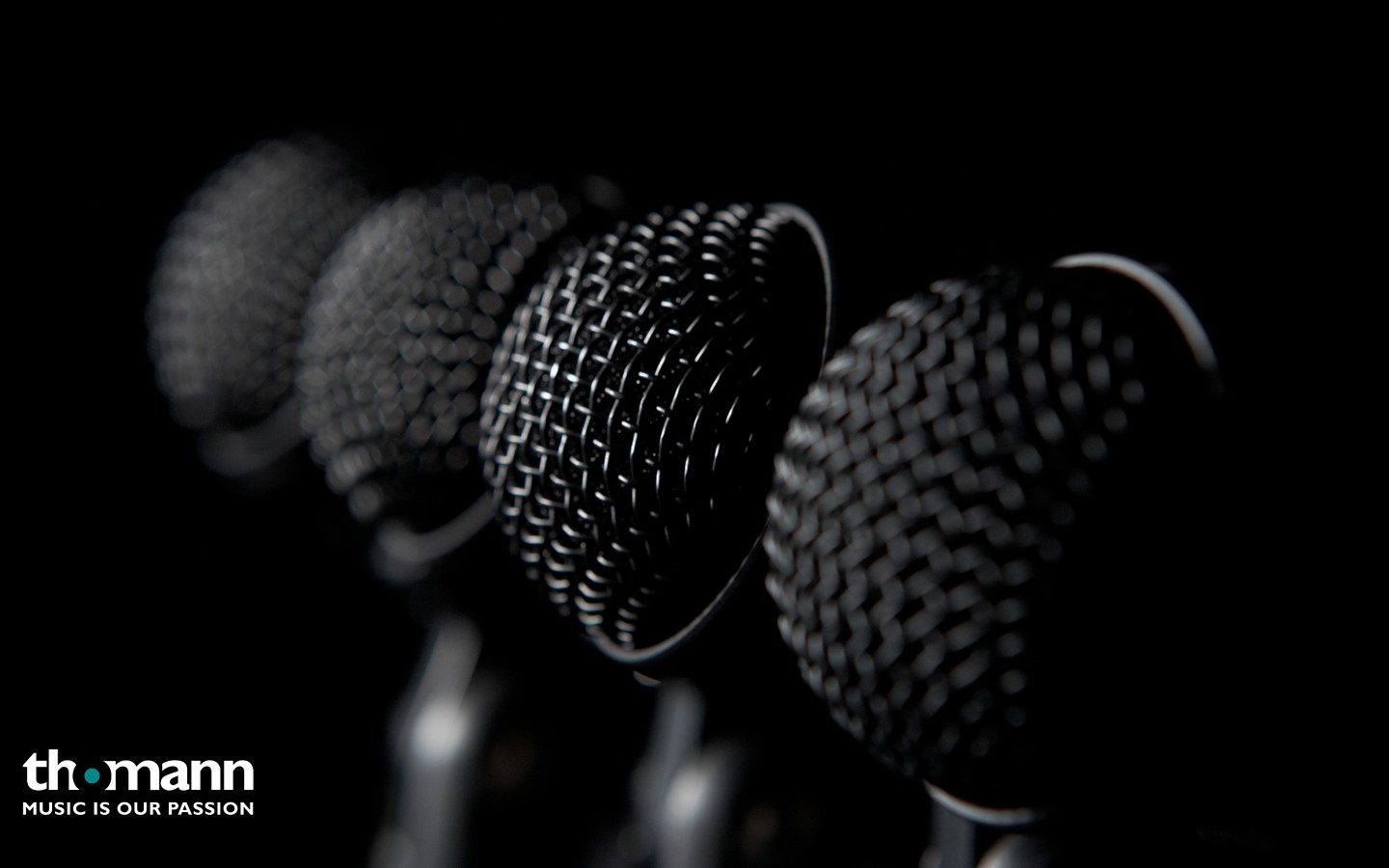This image features a row of four microphones positioned diagonally from the top left to the top right, set against a completely black background. The vibrant black, gray, silver, and blue hues are evident in the image, lending it a sleek, professional appearance. Notably, the second microphone from the left is in crystal-clear focus, while the others progressively blur, with the foremost microphone also slightly out of focus. The microphones, identifiable by their half-circle woven metal grills painted black, are mounted on black mic stands, though only a small portion of the stands is visible. In the bottom-left corner, there is a logo and text, "Thoman - music is our passion," where the 'o' in 'Thoman' features a distinctive design resembling a record: a black circle with an aqua blue dot in the center. The image appears to be a high-quality promotional shot likely intended for Thoman's website, showcasing their range of microphones to potential consumers.